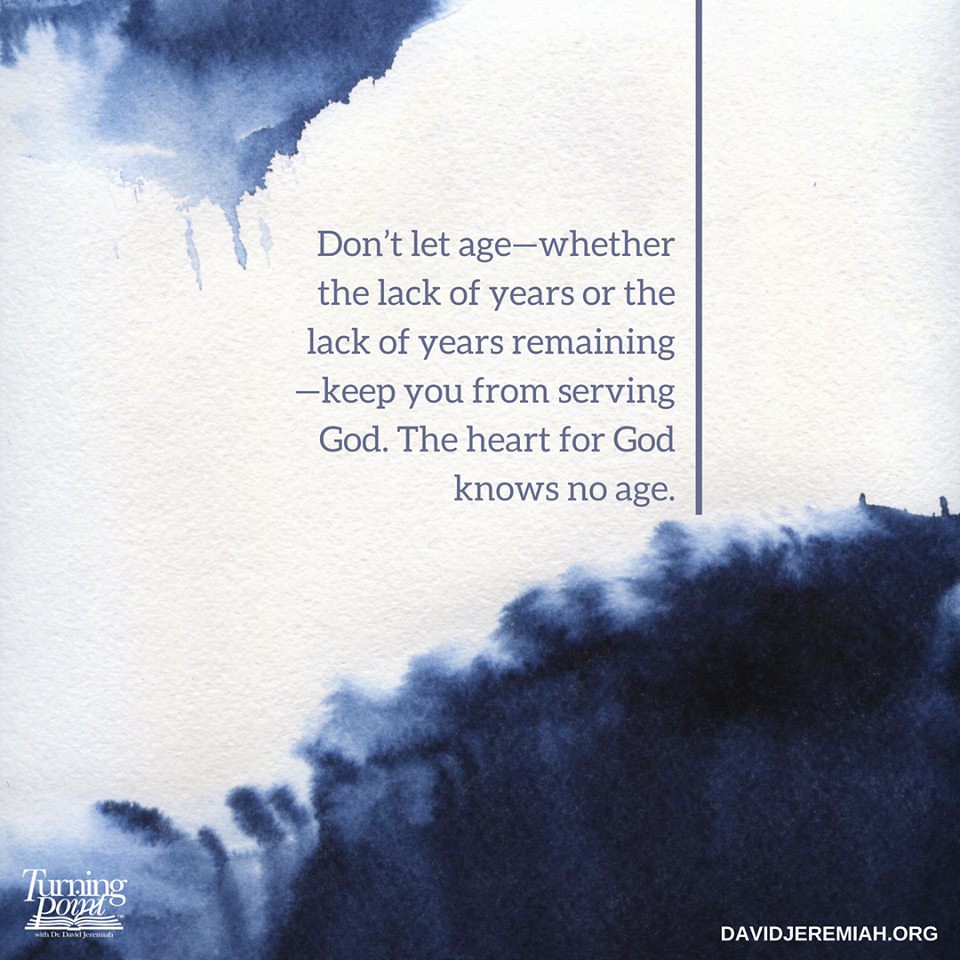This image portrays a textured white paper background featuring artistic splashes of dark blue paint at the upper left and the lower right corners, creating a watercolor effect. The paint drips playfully across the surface, adding an abstract touch. Centrally, in a greyish-blue font, the text reads: "Don't let age, whether the lack of years or the lack of years remaining, keep you from serving God. The heart for God knows no age." A vertical blue line runs from the top of the image to the beginning of the paint at the bottom, adding structure to the design. In the bottom right corner, white capital letters spell out "DavidJeremiah.org," while the bottom left corner features the text "Turning Point" accompanied by a clipart-style open book icon, suggesting this might be a religious pamphlet or inspirational print piece.